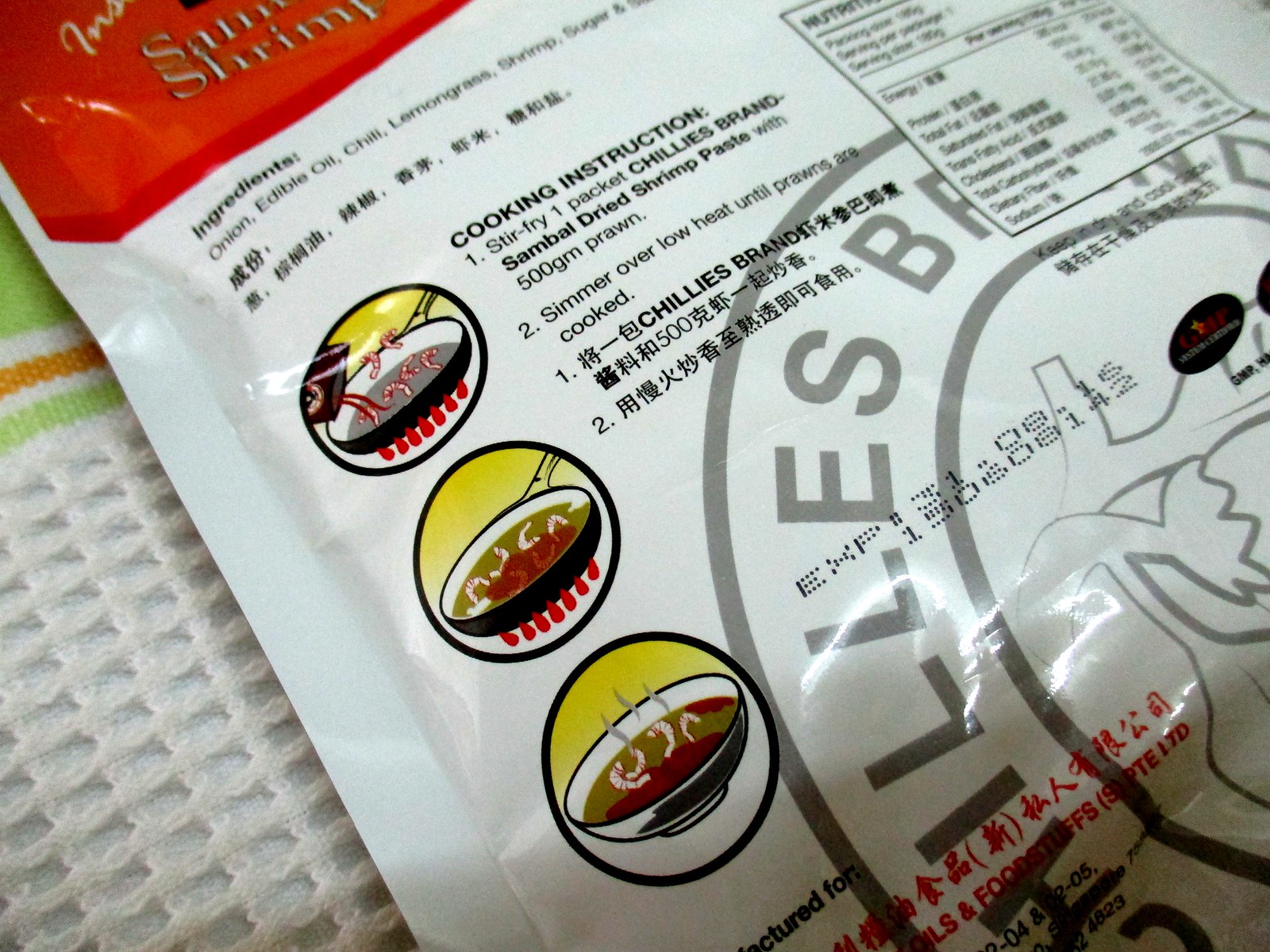The photograph depicts the back of a white packaging bag for Chili's brand sambal dried shrimp paste, prominently featuring cooking instructions and ingredient details. The packaging, accented in red, displays clearly the top-left words "shrimp" alongside instructions primarily in English with some Asian script, likely Chinese. Detailed cooking instructions specify stirring one packet of the sambal dried shrimp paste with 500 grams of prawn, then simmering over low heat until the prawns are cooked. The ingredients listed include onion, edible oil, chili, lemongrass, shrimp, and sugar. Visible nutritional information provides data on calories, total fats, proteins, trans fats, and cholesterol. Illustrated steps next to the instructions depict the paste being poured into a saucepan, stirred, and the finished dish served in a bowl. The package lies on what appears to be a white, green, and orange towel.